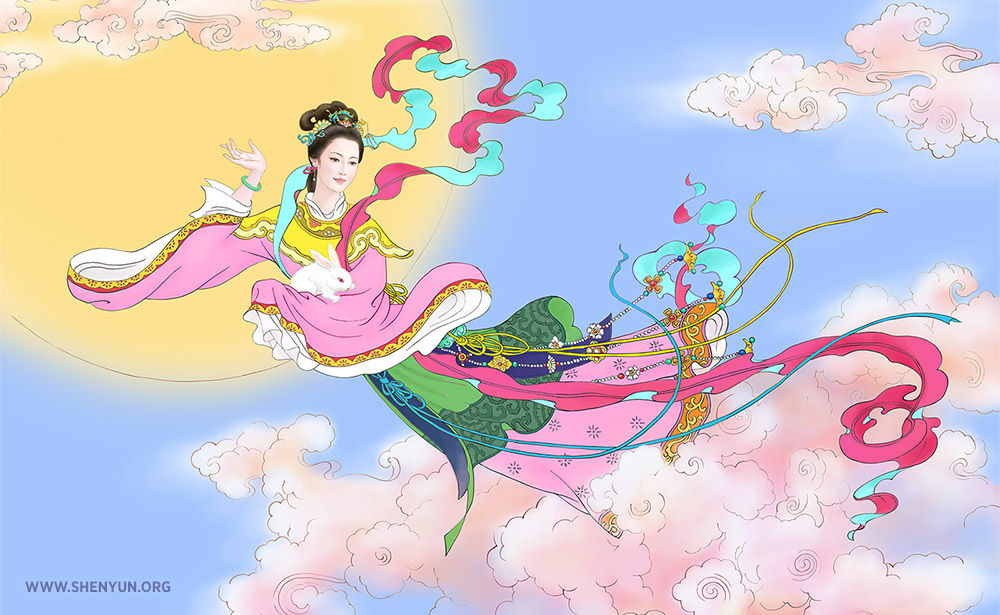The illustration is a colorful, fantasy-inspired depiction of an Asian woman, most likely Chinese, wearing a pink kimono with a long, flowing green dress underneath, which transitions into pink at the bottom. She is floating gracefully above delicate, faint pink clouds in a light blue sky. Spirals of ribbons and scarf-like adornments in shades of pink, red, and teal dance around her in the wind. Her right hand is adorned with a bracelet, and she cradles a rabbit in her left arm. Behind her, the bright yellow sun illuminates the scene from the top left corner, adding a surreal glow. While the drawing has a cartoony feel, the woman's face and arms are rendered with realistic details, creating a contrasting blend of styles. The bottom left corner of the image includes a logo reading "www.shenyang.org," further emphasizing its possible Chinese cultural ties.